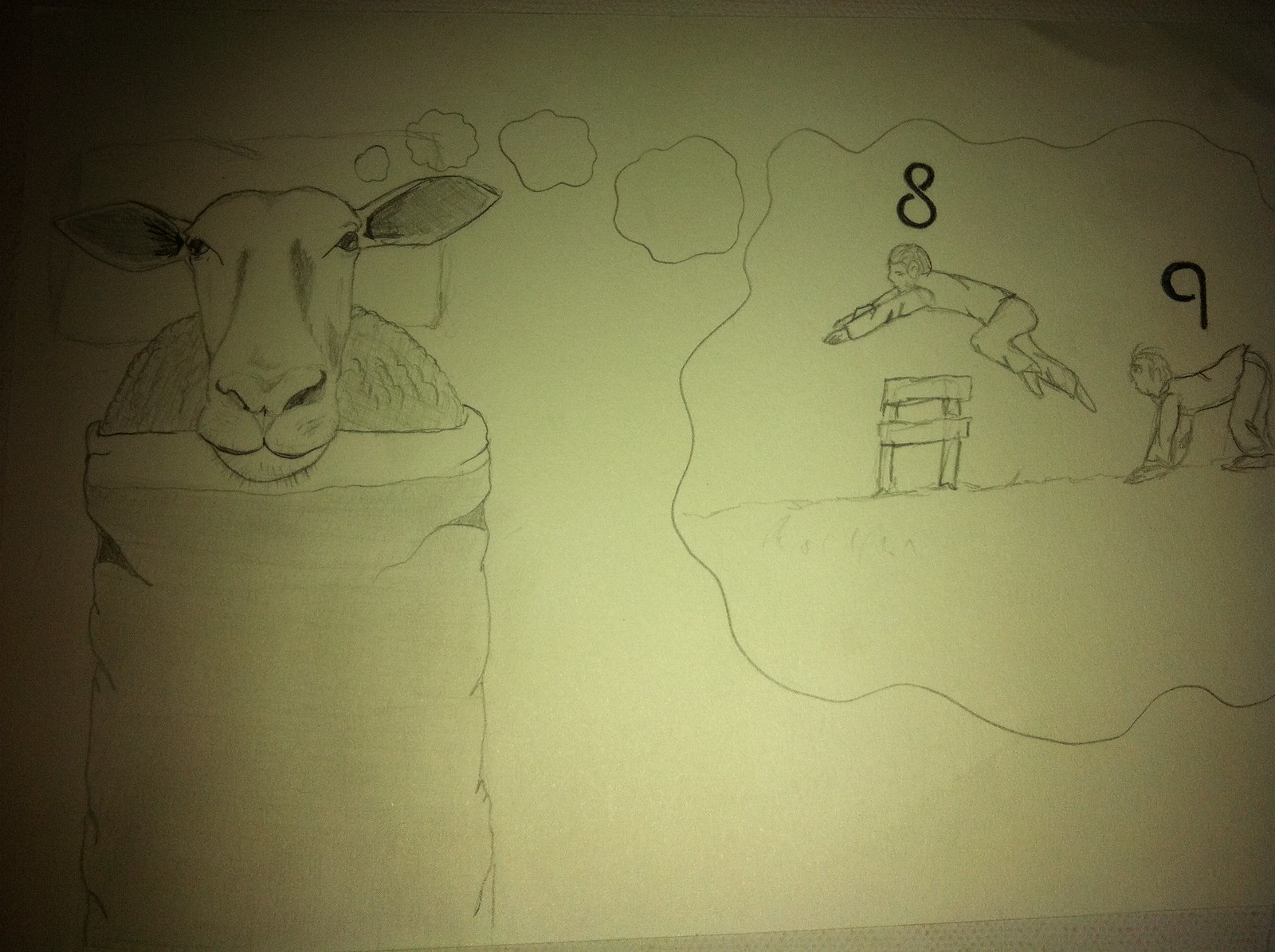This detailed illustration, captured in a photograph, depicts a cow lying in bed under a cozy blanket. The cow, with its large ears and serene expression, rests on a white, rectangular pillow against a white paper background. The monochrome sketch appears to be done with pencil or black ink, and the entire scene is slightly tinged with a yellow hue due to the lighting in the photograph. The cow lies in quiet repose, gazing directly at the viewer.

Extending from the cow’s head are clouds forming a large dream bubble on the right side of the image. Inside this bubble, the dream manifests as two human boys, labeled with the numbers '8' and '9' in dark ink, mimicking a scene of counting sheep to induce sleep. The boys, dressed in shirts and pants, are depicted jumping over a wooden fence, with one boy on all fours waiting as the other leaps. This dream within a dream showcases the whimsical idea of a cow, usually synonymous with restful farm life, counting humans to drift into slumber.